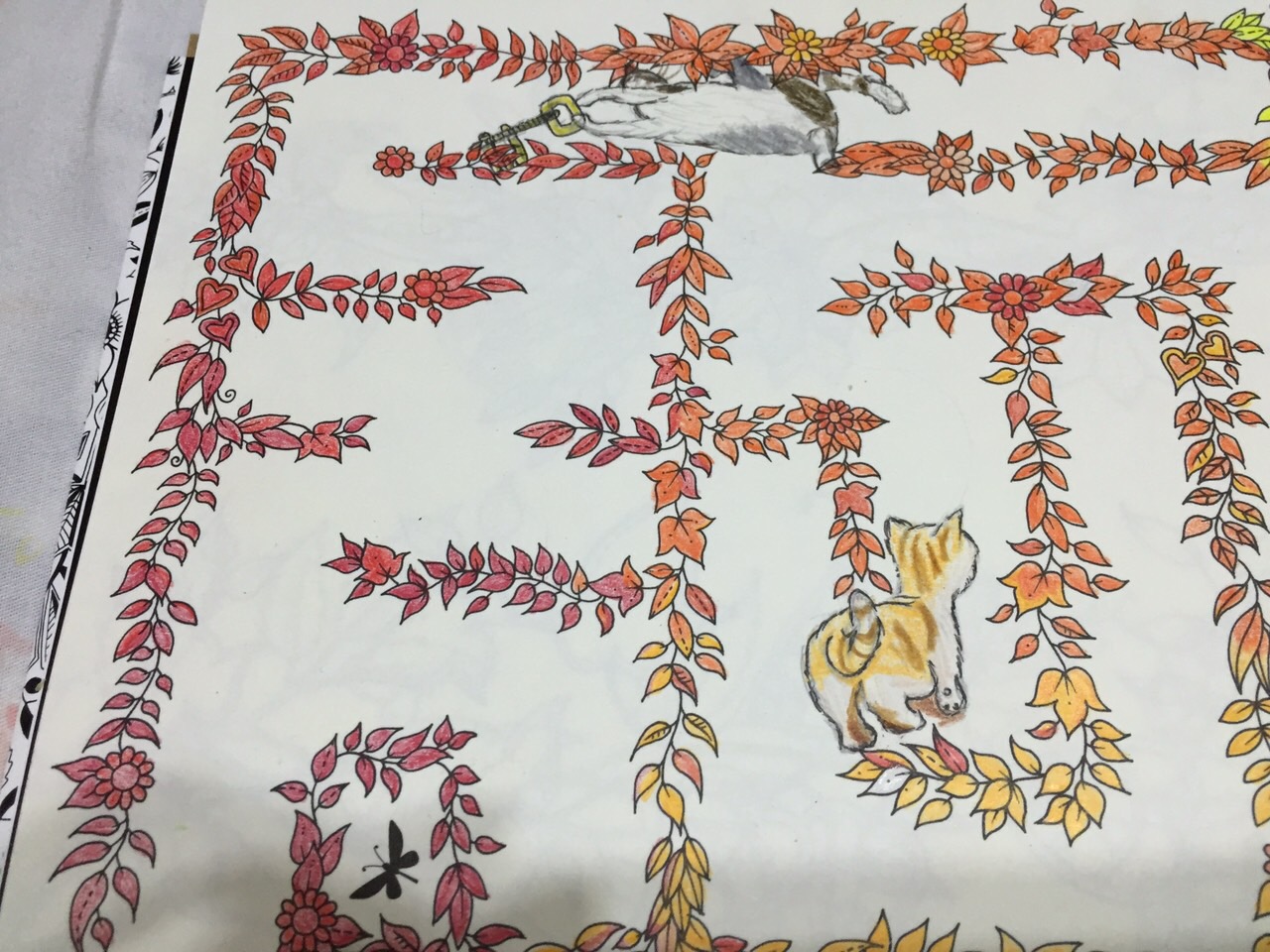The image depicts a page from a coloring book that has been meticulously colored in. The paper, which is white, is placed atop an object showing a black and white binder—suggesting it may be a book or a tablet. The primary design of the coloring page is a maze, with the maze's paths creatively illustrated using leaves and vines. In the center, an adorably drawn orange kitten appears to be just entering the maze. The floral elements around the maze are vividly colored in shades of gold, red, purple, and yellow, adding a vibrant touch to the scene.